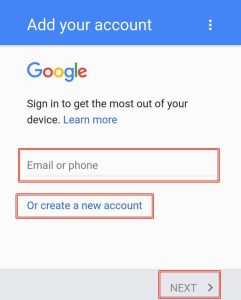The image depicts a sign-in page for a Kukli account, with distinct sections and highlighted elements. The upper portion of the image features a blue background with white text that reads, "Add your Kukli account." To the right of this text is an options icon. 

Beneath this section, the background shifts to white. The word "Kukli" is prominently displayed with each letter in a different color: K is blue, U is red, K is yellow, L is blue, and I is green. Below "Kukli," black text instructs the user to "Sign in to get the most out of your device." Additionally, there is a "Learn more" link in blue text.

Further down, there is a text box labeled for "Email or phone," which is outlined in red, indicating it needs attention or is a required field. Below this, another option reads, "Create a new account," also within a red-outlined box. 

The bottom portion of the image has a grey background. On the bottom right, the word "Next" is displayed within a red-outlined box, indicating the button to proceed. 

Overall, this page is designed for users to enter their email or phone number and press "Next" to continue with signing in or creating a new Kukli account.